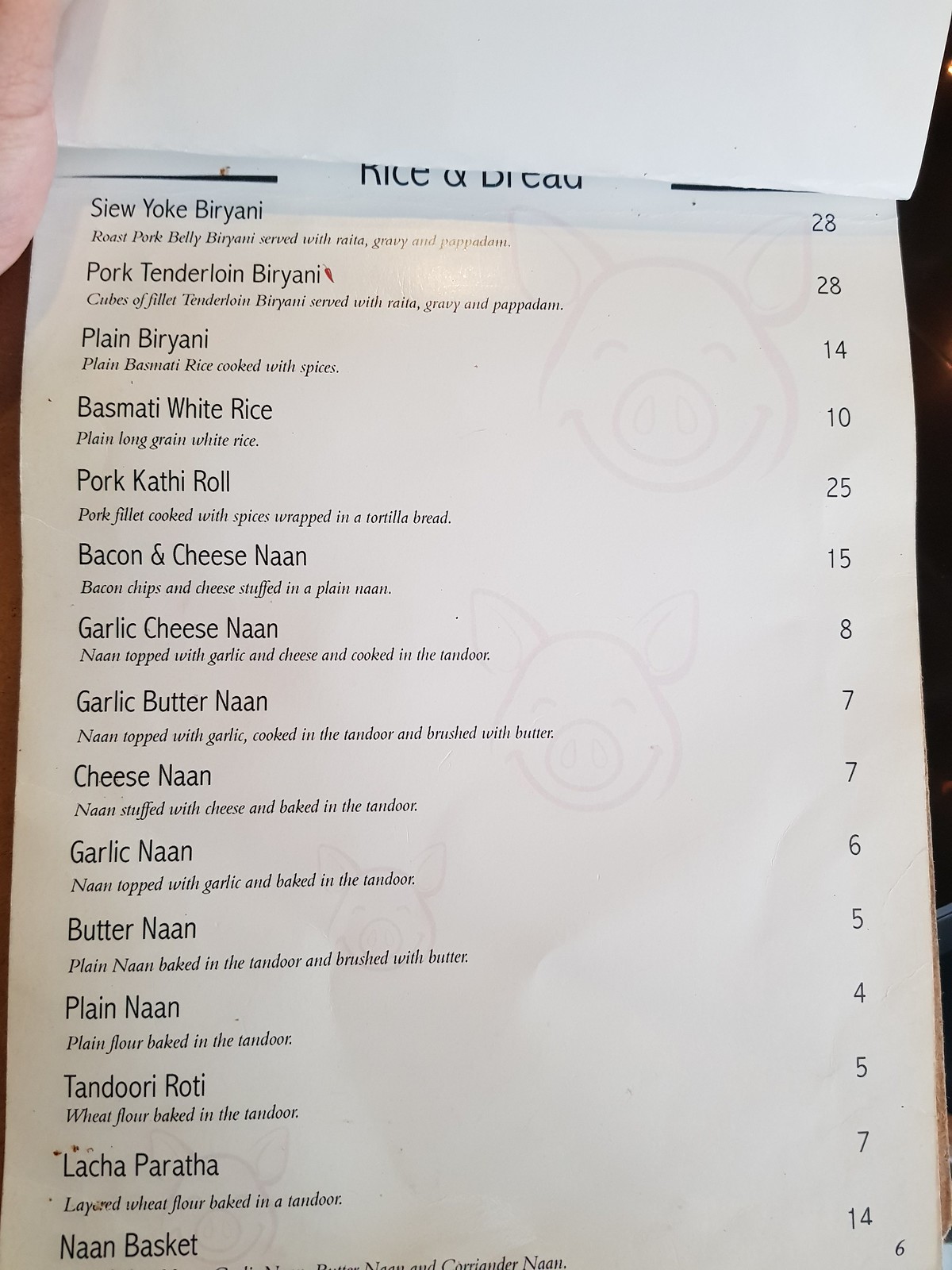This image captures a detailed section of a restaurant menu printed on white paper. The menu items are listed on the left side with their corresponding prices on the right. At the top of the image, partially cut off but still legible, is the heading "Rice and Bread" in bold black text.

Below the heading, the menu features:
- Sayuk Biryani priced at 28.
- Pork Tenderloin Biryani also priced at 28.
- Plain Biryani listed at 14.
- Bismati White Rice priced at 10.
- Pork Kathi Roll, where “Kathi” is spelled K-A-T-H-I, priced at 25.
- Bacon and Cheese Naan priced at 15.
- Garlic Cheese Naan listed at 8.
- Garlic Butter Naan priced at 7.
- Four versions of Naan including Cheese, Garlic, Butter, and Plain, with prices of 7, 6, 5, and 4 respectively.
- Tandoori Roti priced at 5.
- Lacha Paratha listed at 7.
- A Naan Basket at the bottom of the list priced at 14.

The details provide a clear and comprehensive overview of the 'Rice and Bread' section of the menu, highlighting a variety of dishes and their respective prices.